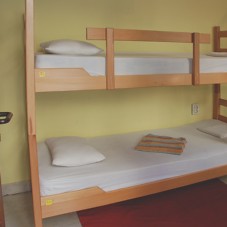This photograph depicts a simple, light wood-framed bunk bed against a pale yellow wall. The beds are sparsely furnished with white sheets and a single white pillow placed on the left side of each mattress. A thin railing composed of three wooden slats is installed on the top bunk to prevent falls. At the foot of the bunk bed, a ladder made from the same light wood serves as the means to access the top bunk. Noticeable in the room, the bottom bunk has a multi-colored blanket folded neatly in a small square, featuring hues of orange, red, blue, and yellow. The floor is covered in dark brown wood, accentuated by brown crown molding and a maroon rug. Visible in the background is a partially cut-off door handle on the left side of the image. The room appears quite stark and unadorned, likely intended for temporary accommodation. The overall ambiance feels cold and barren, with minimal furnishings contributing to a sense of austerity.